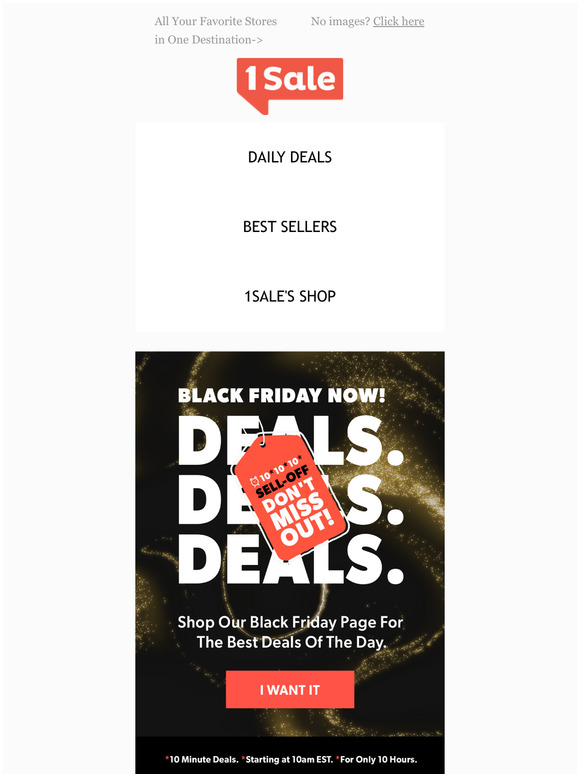The image features a predominantly cream white background with grayish tones along the left and right sides, extending vertically down the frame. Centered at the top, the text "All your favorite stores in one destination" is written in gray, accompanied by a small arrow pointing to the right.

To the right, centrally located, there is a message indicating "No images, click here," with the phrase "click here" underlined, suggesting it functions as a clickable button.

An orange speech bubble is positioned prominently, stating "1" in white, highlighting a "Number One Sale." Below this, vertically aligned black text reads "Daily Deals, Best Sellers, One Sale Shop."

An illustration resembling an evergreen tree or Christmas ornament bears white text that says "Black Friday now, Deals, Deals, Deals." Superimposed on these words is a red sales tag announcing "10% off, don't miss out" with the text "sell off" in black.

Further down, white text encourages viewers to "Shop our Black Friday deals page for the best deals of the day." A red button with white text urges, "I want," followed by a note at the bottom indicating "10-minute deals starting at 10 a.m. EST, only for 10 hours."